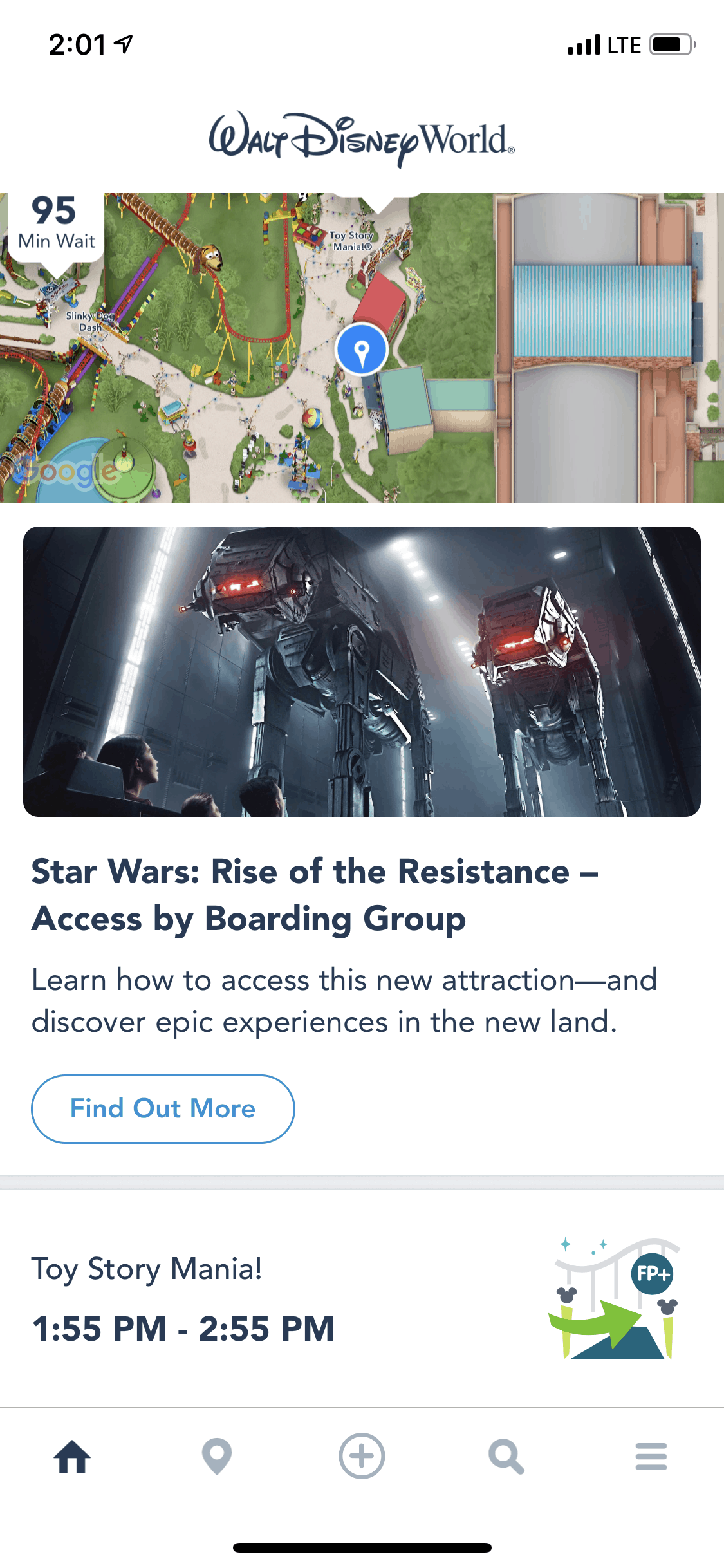In this detailed screenshot, we observe the interface of either a tablet or a cell phone. The upper left corner displays the time as 2:01, accompanied by a small arrow pointing northeast. To the right of this, there is an LTE icon alongside four signal bars, indicating strong network reception. Additionally, a battery icon shows approximately 75% charge.

Beneath these status indicators, the text reads "Walt Disney World," signifying the theme of the content displayed. Below this heading, a detailed map of a segment of a theme park is visible. The map features areas of grass, several rides, and an indication of a 95-minute wait time for a particular attraction. A notable blue location icon suggests the current location of the user on the map.

Further down the image, a promotional picture for a Star Wars attraction is present. It features mechanical structures recognizable from Star Wars lore, specifically the AT-AT Walkers, though they are referred to as "Star Walkers" in the description. Below this visual, text reads: "Star Wars: Rise of the Resistance. Access by boarding group. Learn how to access this new attraction and discover epic experiences in the new land." Accompanying this text is a button labeled "Find out more."

Following this, there is scheduling information for "Toy Story Mania," showing an available window from 1:55 p.m. to 2:55 p.m. Adjacent to this information is a green highlighted area.

At the screen's bottom, there is a navigation bar containing icons for home, location, adding new items (represented by a plus button), searching (represented by a magnifying glass), and a menu (depicted by three horizontal lines).